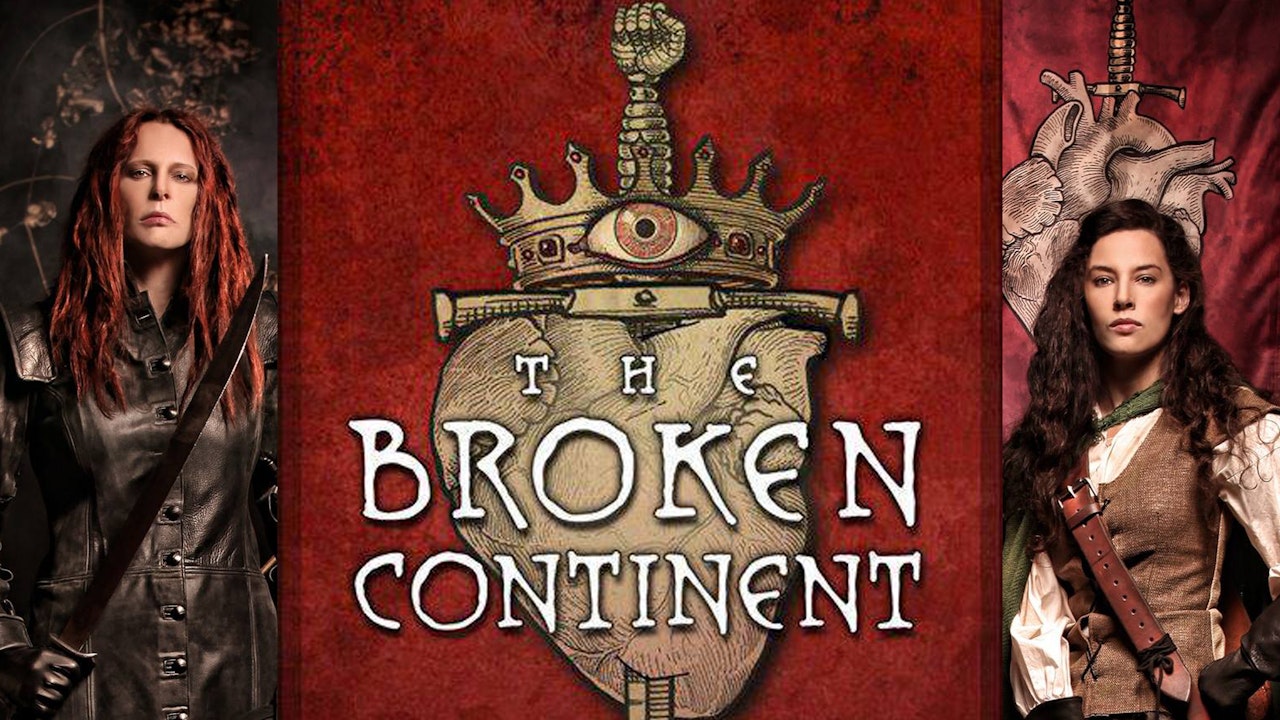In the center of the image stands a striking red board, serving as a backdrop for an intricate emblem. Atop the emblem sits a crown featuring a single eye, from which a lower arm extends outward. Below the crown, a shawl is draped horizontally, followed by the shape of a heart. This entire detailed logo is rendered in a light brownish-grey hue. Above the emblem, the phrase "The Broken Continent" is prominently displayed in white.

On the left side of the red board, a woman with long red hair—styled in dreads—stands confidently, holding an upright sword. She is dressed in a long black leather coat and is set against a dark grey background with dead brown leaves strewn behind her.

On the right side, another woman gazes directly at the camera with a serious expression. She has long, curly brown hair and is clad in a white t-shirt layered with a brown vest, reminiscent of Robin Hood attire, complete with a green sash across her shoulder. Her backdrop is a reddish-maroon cloth with a depiction of a heart pierced by a knife.

Both women have intense, captivating presences, enhancing the dramatic and evocative atmosphere of the image. The contrasting backgrounds and the detailed, symbolic emblem centralize the theme of "The Broken Continent," reinforcing the overall narrative and artistic composition.